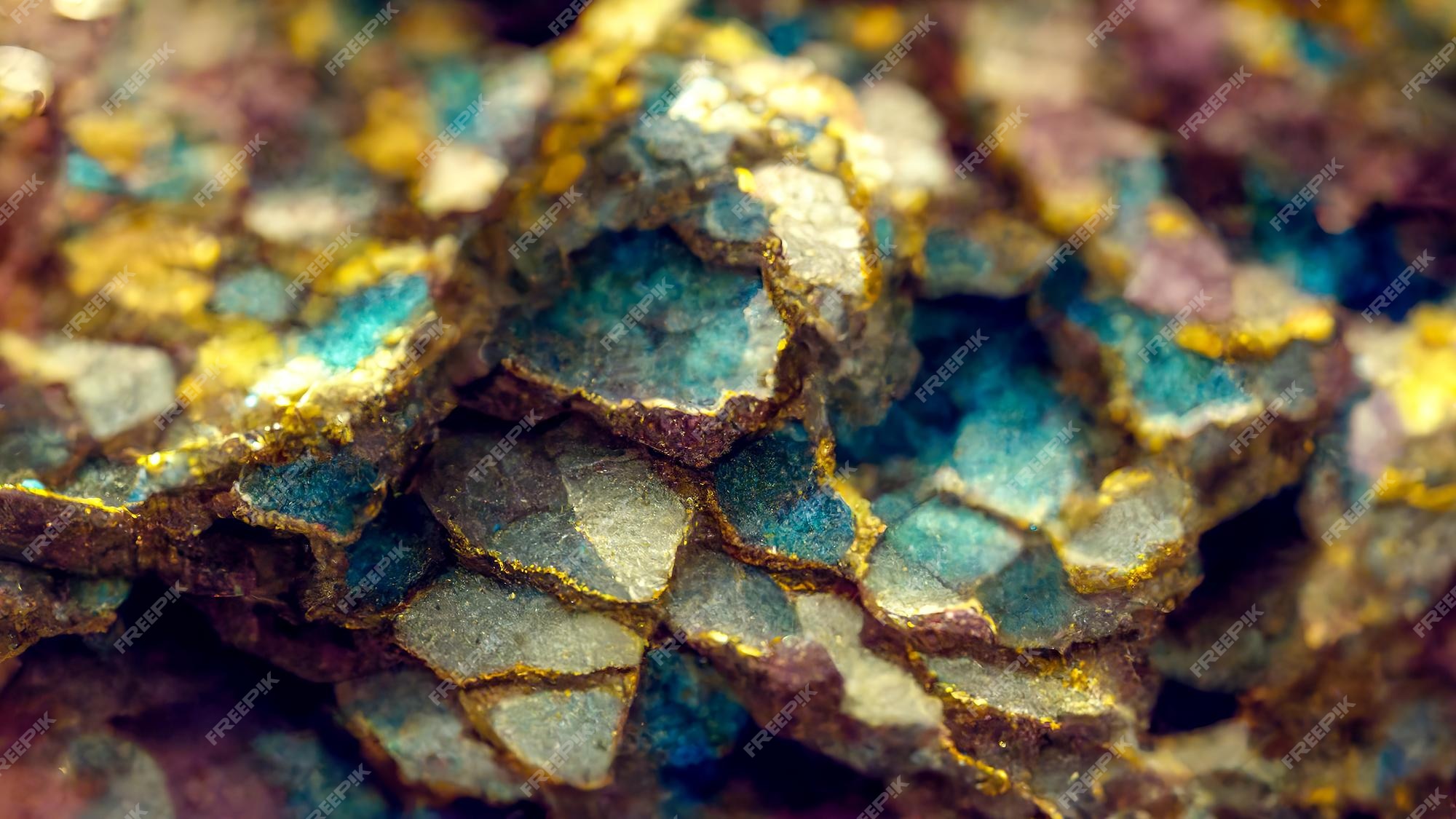This image is a detailed 3D rendering, rectangular in shape with the top and bottom sides being twice as long as the left and right sides. It primarily features a close-up of multi-cracked stone surfaces that exhibit a myriad of vibrant colors, including shades of blue, purple, aqua, and white. Intricate golden edges outline these cracks, resembling fine gold dust or glitter, giving the impression of either scales, tiles, or even layered crystals. Adding to the textured richness of the image, there is a semi-transparent white watermark that repeats diagonally across the photograph. The watermark reads FREEPIK, where the letter "i" is stylized as an exclamation mark, hinting that this might be sourced from a stock image marketplace. The watermark, while noticeable, is subtly integrated into the background, ensuring it doesn't overpower the visual details of the richly colored and gold-accented stone textures.